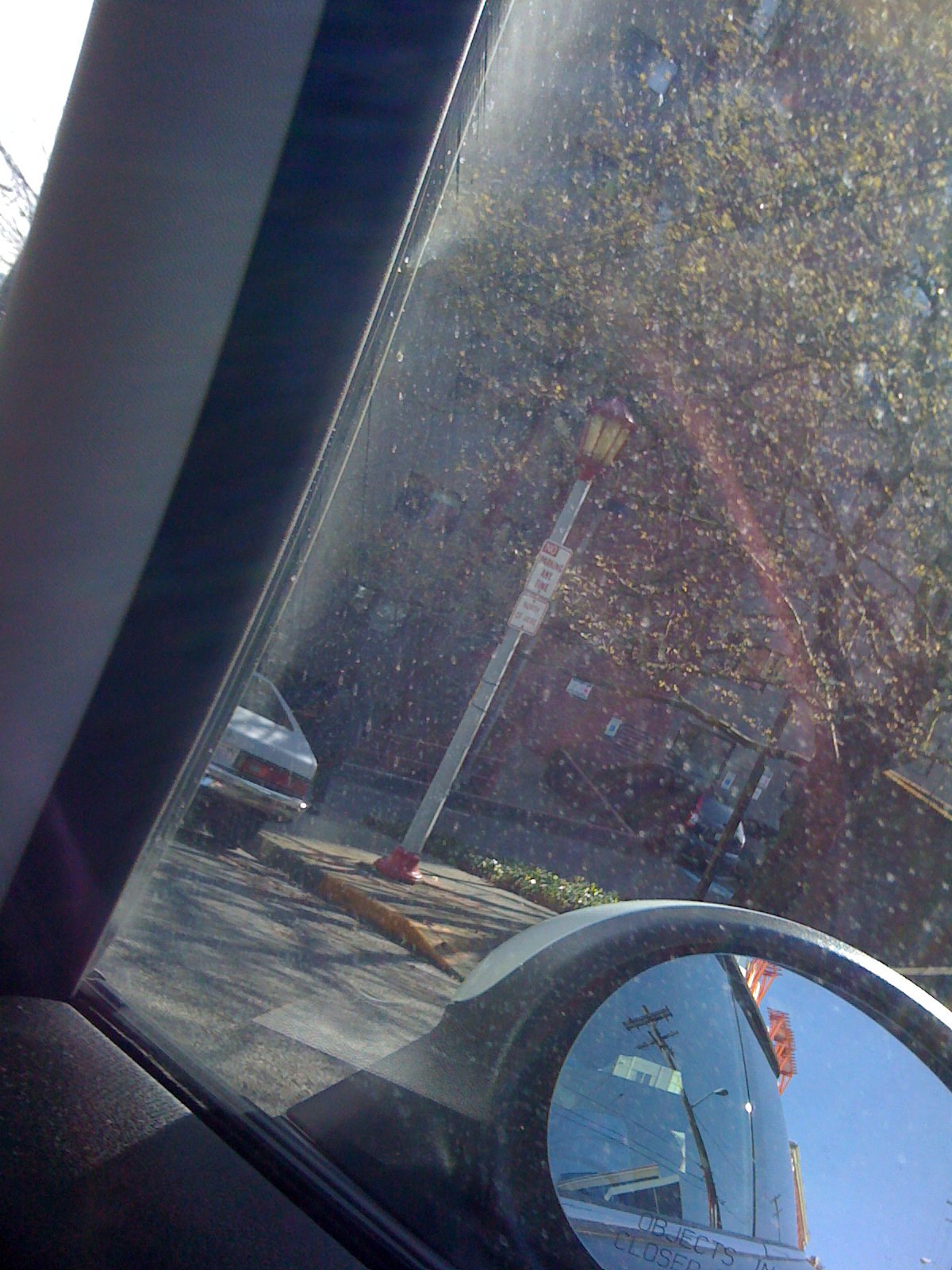Captured from within the interior of a car, this photograph showcases a tilted, portrait-oriented view through the window. The car's rear and side mirrors are visible, with the side mirror reflecting part of the vehicle, revealing its flat exterior. Notably, headlights or other roof-mounted lights suggest it could be a law enforcement vehicle. Outside the vehicle, a tree is shedding its leaves, indicating the onset of fall. A small white car is parked at the corner, accompanied by a vintage lantern-style streetlight mounted on a metal pole, which also features a sign. The background includes several buildings, completing the urban scene.